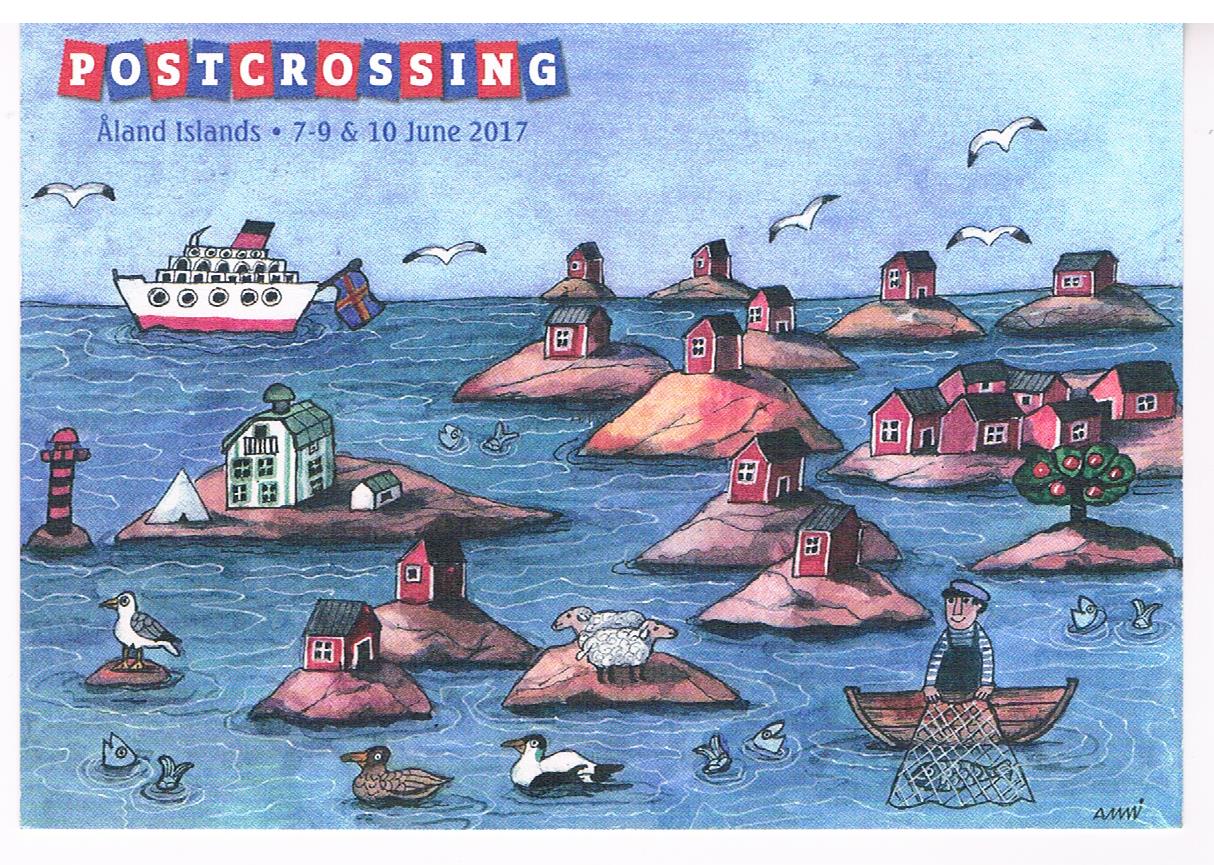The image depicts an old-school cartoon-style advertisement showcasing a picturesque, idyllic archipelago. The scene features an array of small islands, each adorned with various elements. Dominantly, the islands host single-story red huts with black roofs, creating a charming, rustic vibe. On "Old Smile Island," clusters of these huts are visible, enhancing the quaint atmosphere.

In the foreground, a man in a striped shirt is fishing from a small boat, skillfully pulling fish from the water. Surrounding him, a lively marine scene unfolds with fish jumping out of the water and birds either skimming the surface or perched nearby. A couple of sheep graze on another island, while a mound with a tree bearing red fruit adds a touch of natural beauty.

To the top left, a boat—potentially flying a flag resembling the Danish flag—sails off into the distance. The skies are dotted with birds, some soaring above the horizon, establishing a sense of peaceful movement. 

Overlaying this charming tableau is text in white letters, set against alternating red and blue backgrounds, spelling out "Postcrossing" at the top. Below this, there’s an inscription indicating "Åland Islands, 7th to 9th, 10th June 2017," also located in the top left-hand corner. This meticulous detail and the vintage aesthetics make the image feel like a nostalgic yet vibrant ad illustration.